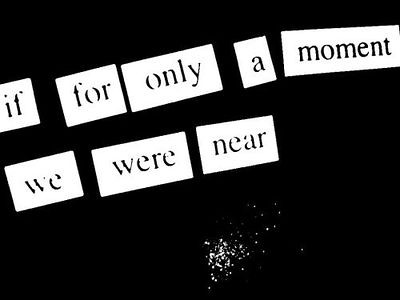The image features a predominantly black poster adorned with rectangular white patches. These patches, which appear to resemble paper cutouts or magnet word art, each contain a single black word, collectively spelling out the phrase "if for only a moment we were near." The words are arranged from the upper left to the upper right, and then from the center left to the center right. Below this textual arrangement, the bottom center of the poster showcases an array of white speckles that diffuse and taper off as they ascend, adding a subtle decorative element. The stark contrast between the black background and the white text and patches creates a visually striking, minimalist composition.